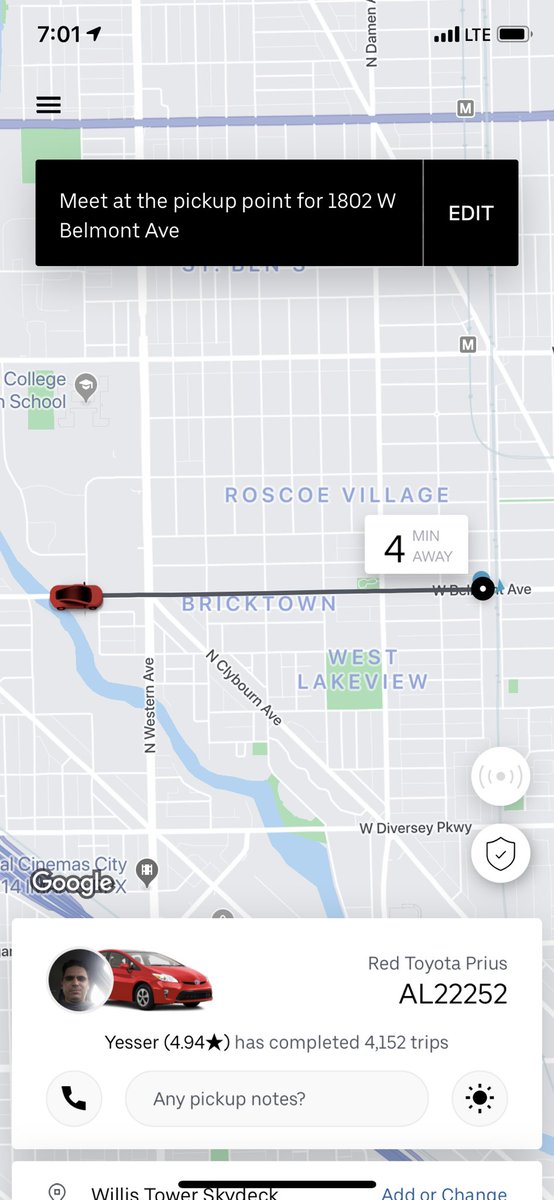Here's a detailed and cleaned-up caption for the image:

"This is a screenshot of a rideshare app displayed on a smartphone. The background features a grid-style map from Google Maps, where streets are depicted in white and blocks in gray. To the left side of the map is a small river flowing from the middle toward the bottom. Prominent neighborhood labels on the map include Roscoe Village, Bricktown, and West Lake View. 

In the top-left corner of the screenshot, the time '7:01' is displayed in black text, accompanied by a directional arrow pointing up to the right. Below that, there are three horizontal lines stacked vertically. In the top-right corner, connectivity bars, an 'LTE' label, and a battery icon are visible.

Directly beneath this toolbar, a black rectangle contains white text instructing the user to 'Meet at the pickup point for 1802 West Belmont Avenue.' Adjacent to this text is a black button labeled 'Edit' in white text.

The map shows a small red car icon indicating that the ride is four minutes away. At the bottom left of the screen, the Google emblem is displayed. Below this, in a white rectangle, the details of the driver and vehicle are provided. The image reveals a photo of the driver, a man with brown skin, dark hair, and dark eyes. Next to his photo, the text states he drives a red Toyota Prius with the tag number AL2252, and has completed 4,152 trips."